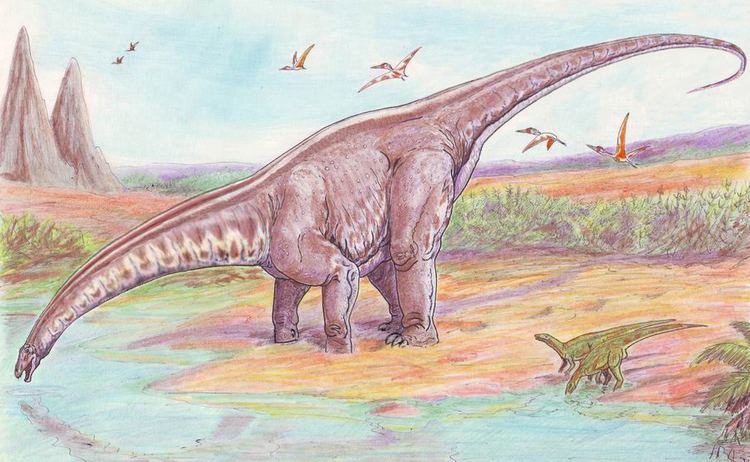The image showcases a detailed and vivid cartoon drawing of dinosaurs in a prehistoric landscape. Central to the scene is a massive brontosaurus with a grayish-brown hue, featuring an impressively long neck and an equally elongated tail that curves upwards to the right. This majestic dinosaur is depicted bending down and reaching forward to drink water from a creek located at the bottom left corner of the image. Its reflection shimmers in the water below.

Adjacent to the brontosaurus, on the right side, are two much smaller green dinosaurs, likely theropods, standing on their hind legs with diminutive front arms. One of these smaller dinosaurs is also bending down to drink from the creek, while the other looks upward at the brontosaurus.

The sky above is a tranquil blue, adorned with scattered, hazy white clouds. Soaring high in the sky are six red and white pterodactyls, adding a dynamic sense of movement to the scene. In the distant background on the left, towering, jagged mountain peaks stand out prominently against the partly cloudy sky. The landscape transitions from these steep mountains to a relatively flat terrain with sparse green vegetation and some bushes lining from the center to the right edge of the image. This picturesque prehistoric tableau is filled with intricate details, illustrating a serene yet lively moment in an ancient world.